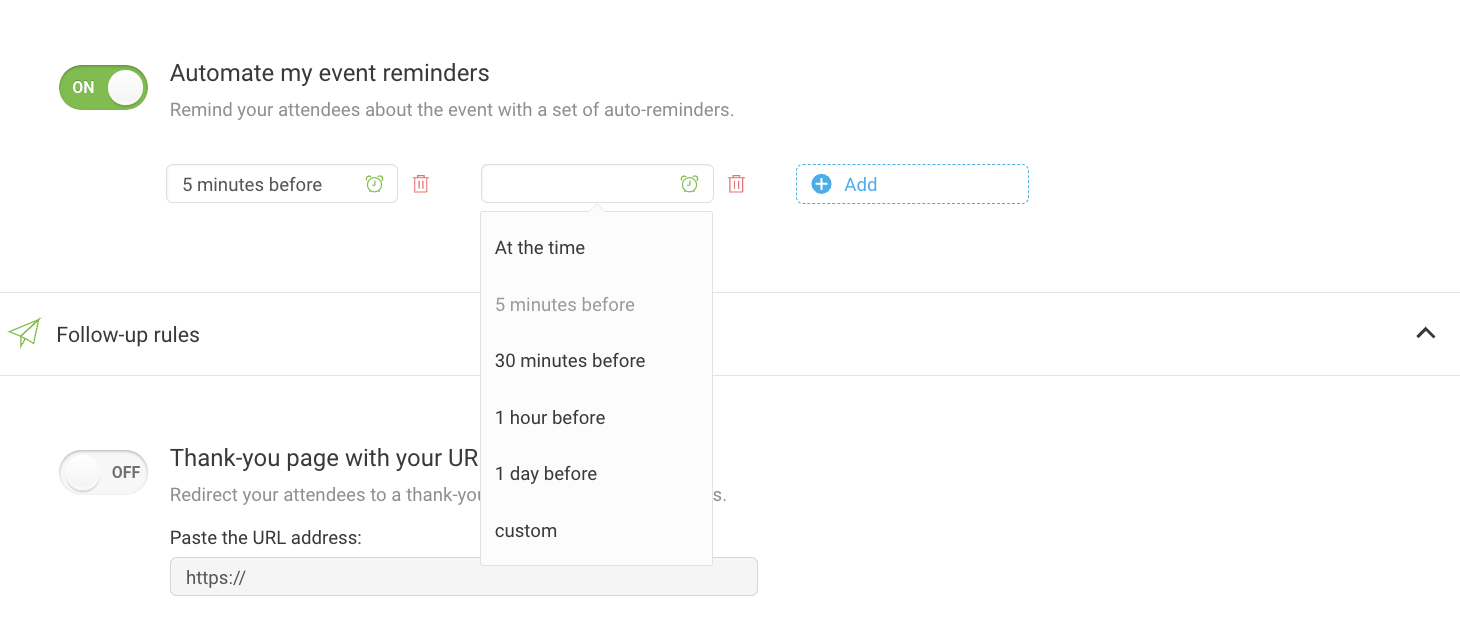In the top left corner, there is a long horizontal green circle with text on one side and a white circle on the other. To the right of this, there is a heading that says "Automate My Event Reminders." Below this heading, a subtext reads, "Remind your attendees about the event with a set of auto reminders."

Beneath this description is a long rectangular area containing the text "Five minutes before." To the right of this text is another empty rectangle, followed by a blue outlined rectangle with a blue circle inside that contains a plus symbol. Next to this is the word "Add," also in blue.

Below this section, to the left, is the title "Follow Up Rules" accompanied by an image of a small green triangle to its left. A list of reminder timings follows: "Five minutes before" in lighter gray text, "30 minutes before" in black text, "One hour before," "One day before," and "Custom."

To the left of this list is a section titled "Thank You Page" with "URL" capitalized. Below this title is the text, "Redirect your attendees to a Thank You page." Underneath this, there is an instruction to paste the URL address, with "URL" again in capital letters. Below that is a box designated for entering an address, containing placeholder text that reads "https://".